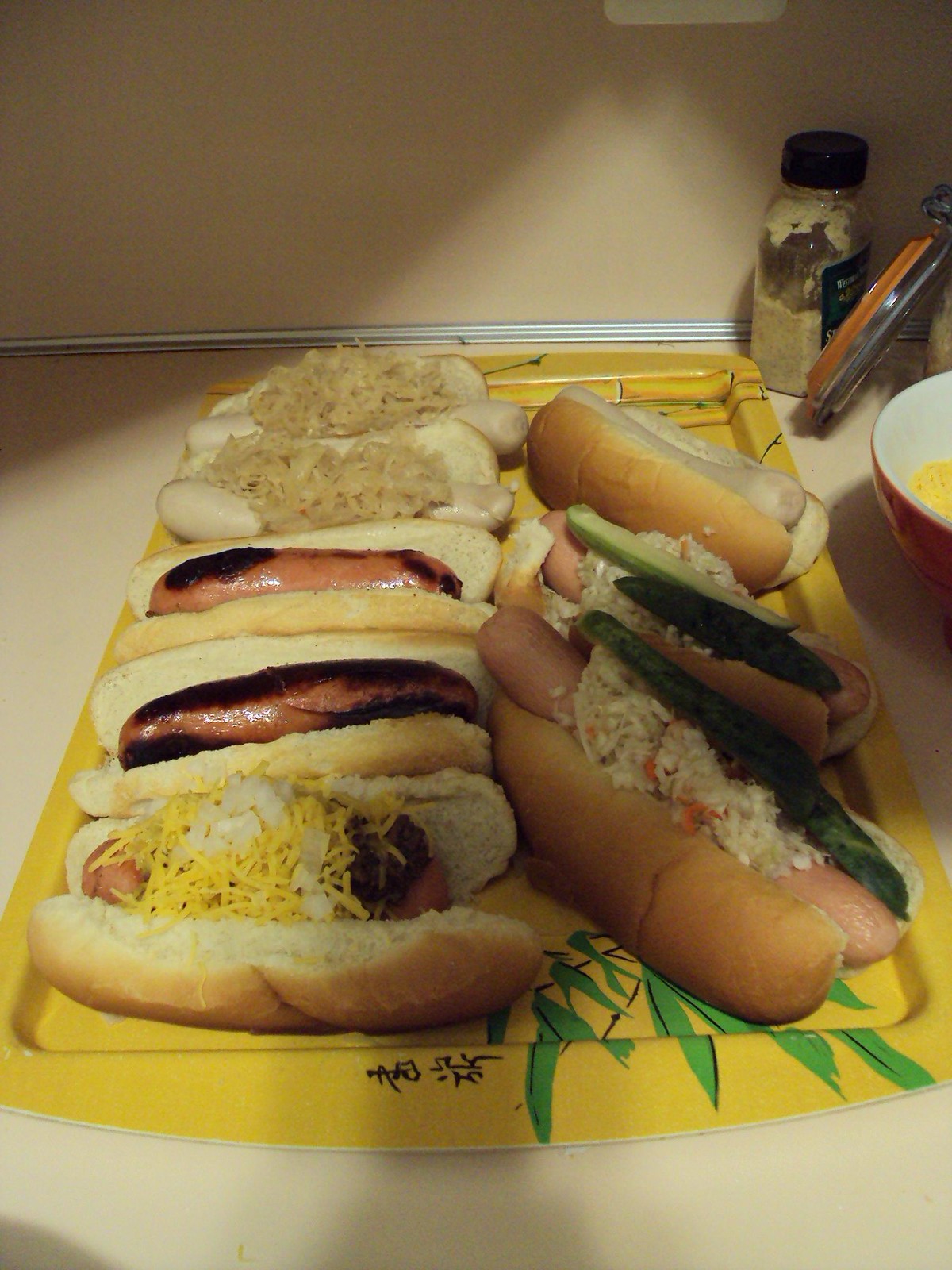The photograph showcases a large yellow tray adorned with green bamboo art and Chinese writing, placed on a beige countertop with a beige backsplash. The tray holds eight hot dogs, each with distinct toppings and variations. At the far end of the tray, two lighter-colored sausages, almost white, are topped with sauerkraut, while another appears plain in a bun. The three hot dogs at the bottom left are clearly grilled, with charred edges; two of these are undressed, and the other is garnished with cheese and onions. Towards the mid to bottom right of the tray, there are two hot dogs dressed with coleslaw and pickle wedges. In the background, a jar of mustard and a dish with various sauces are visible, adding context to this diverse display of hot dogs.